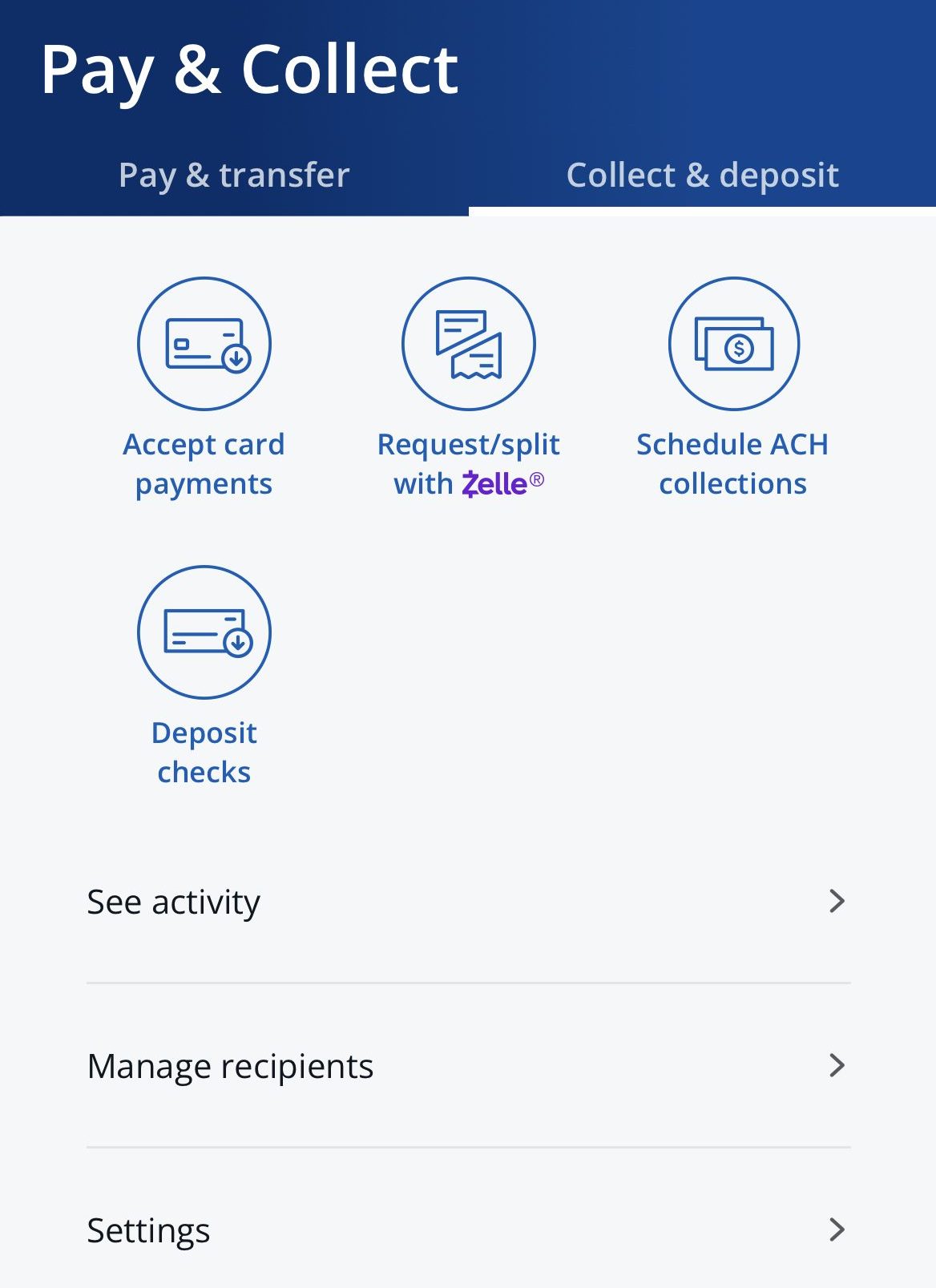This is a screenshot from the Zelle app, an application widely used for sending and collecting money. The interface features a structured layout designed to facilitate various financial transactions. At the top of the screen, a blue banner prominently displays bold white text reading "Pay & Collect." Directly below, in a gray unbolded font, are the options "Pay & Transfer" on the left and "Collect and Deposit" on the right.

The main section of the display presents four circular icons organized in a grid. The top row contains three circles, while the second row features a single circle. 

- The first circle in the top row features an image of a credit card with a downward arrow in the bottom right corner. Below it is the text "Accept Card Payments."
- The middle circle displays an icon of a torn piece of paper, labeled "Request Split," and includes the Zelle logo in purple with a registered trademark (®) symbol.
- The rightmost circle on the top row depicts two dollar bills with a dollar sign and a circle icon, accompanied by the text "Schedule ACH Collections."

In the second row, there is one circular icon featuring an envelope with a downward arrow in the bottom right corner, labeled "Deposit Checks."

Below these icons, the app interface continues with three rows, each containing a single item:
- The first row displays "See Activity" with a right-pointing arrow.
- The second row reads "Manage Recipients," also with a right-pointing arrow.
- The third row shows "Settings," similarly accompanied by a right-pointing arrow.

This structured layout ensures users can quickly navigate and select their desired financial transaction options.